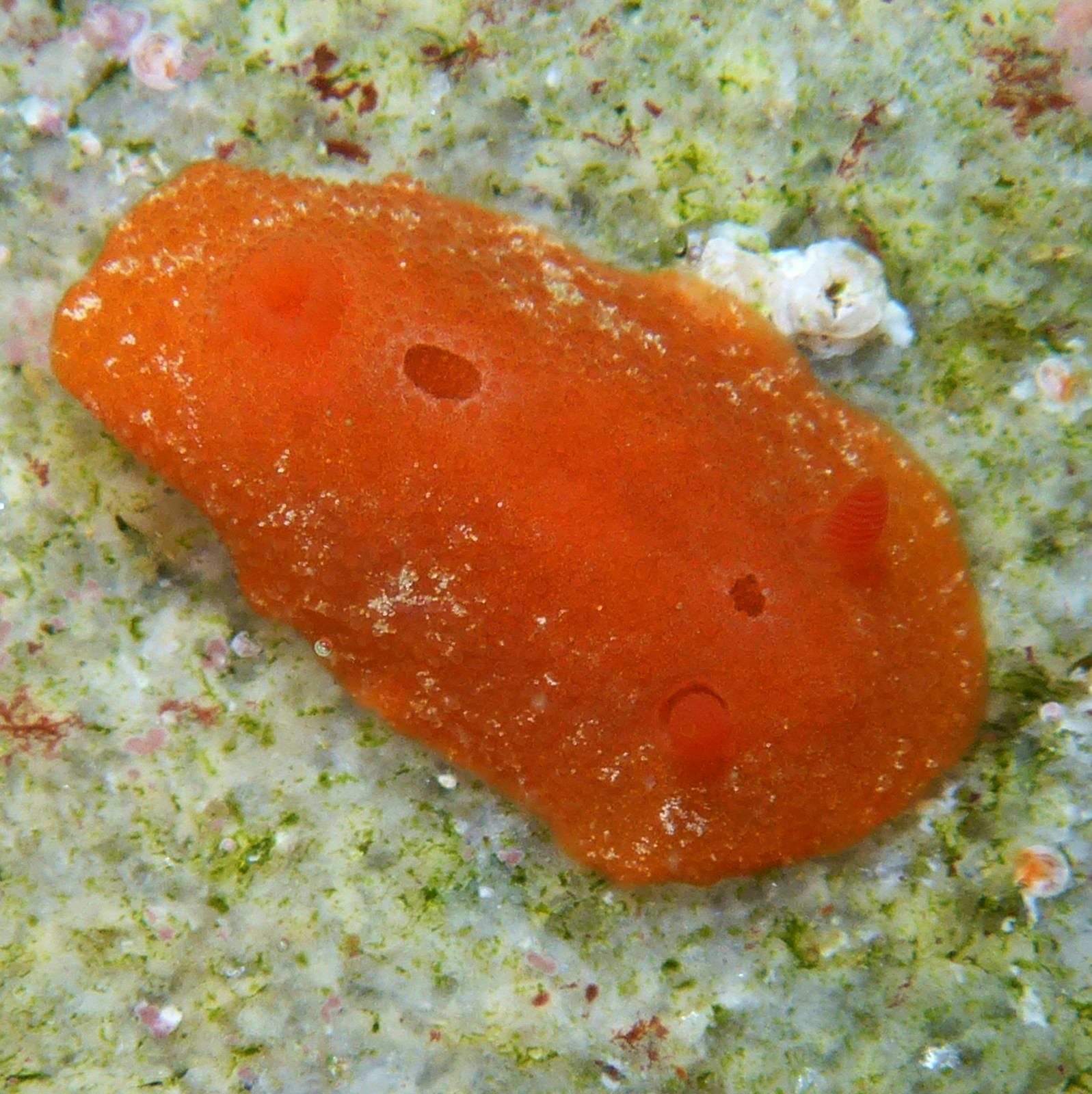The photo captures an oblong orange organism resembling a sea creature or some form of marine lichen, centered within the image. This nondescript blob is detailed with crystal-like granulations and projections that suggest the surface is textured, almost appearing as though small tree-like structures are emerging from it. The creature's oval shape is emphasized with a few indents, and to the upper right, it features a small cone-like protrusion which might be mistaken for an eye, though it's the same color as the rest of the organism.

Surrounding the orange organism is a mixed background, likely within a fish tank environment. The bed it rests upon is composed of white and light green particles, which resemble a blend of sand, crystals, and potentially organic material. The scene includes sporadic red and pink flecks, predominantly concentrated towards the upper left corner, and a noticeable yellow object positioned on the right side behind the organism. The entire backdrop is sprinkled with green and white specks that contribute to the underwater ambiance, suggesting this could indeed be a marine habitat.